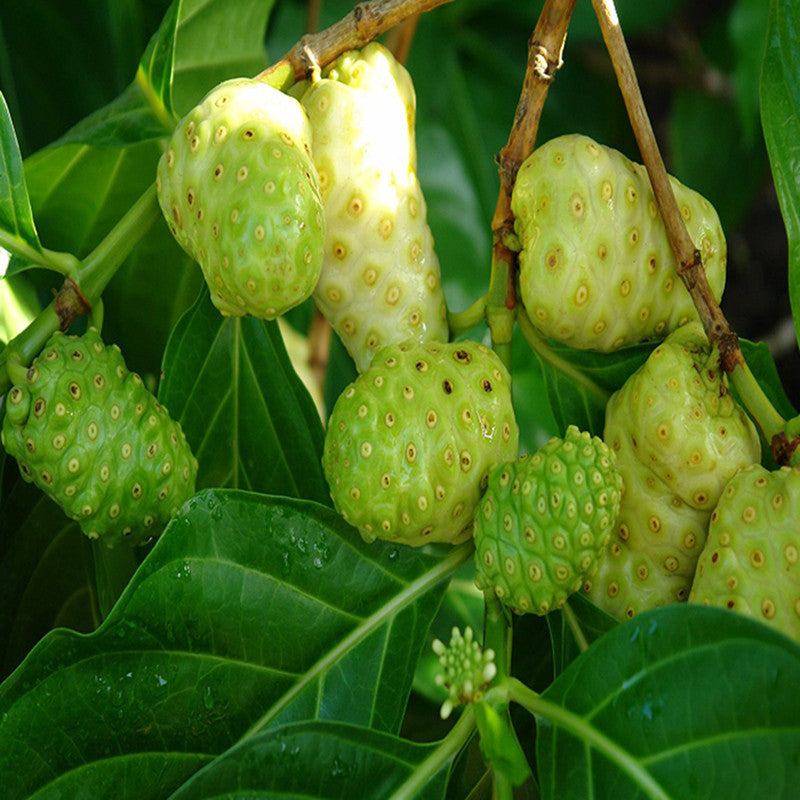The photograph captures a detailed close-up of lush foliage with wet, green leaves and nodules resembling fruits. The leaves are smooth and edged, featuring a distinctive yellow lining and veining against the darker green backdrop. Water droplets cling to the leaves, suggesting recent rain or dew. The branches, rich brown and wooden, stretch from the top of the frame. The fruits themselves are irregularly shaped, adorned with nodules and circular spots in shades of yellow, brown, and green. Some fruits appear vibrant green, while others transition to a paler cream color as they ripen, often developing deep creases and varied surface colors. The odd-shaped fruits range from round to oblong, some even resembling tiny pineapples or prickled pears. The image showcases different stages of the fruit growth, from small buds ready to blossom to more mature forms with nodules and pale speckles, hinting at their tropical origins.